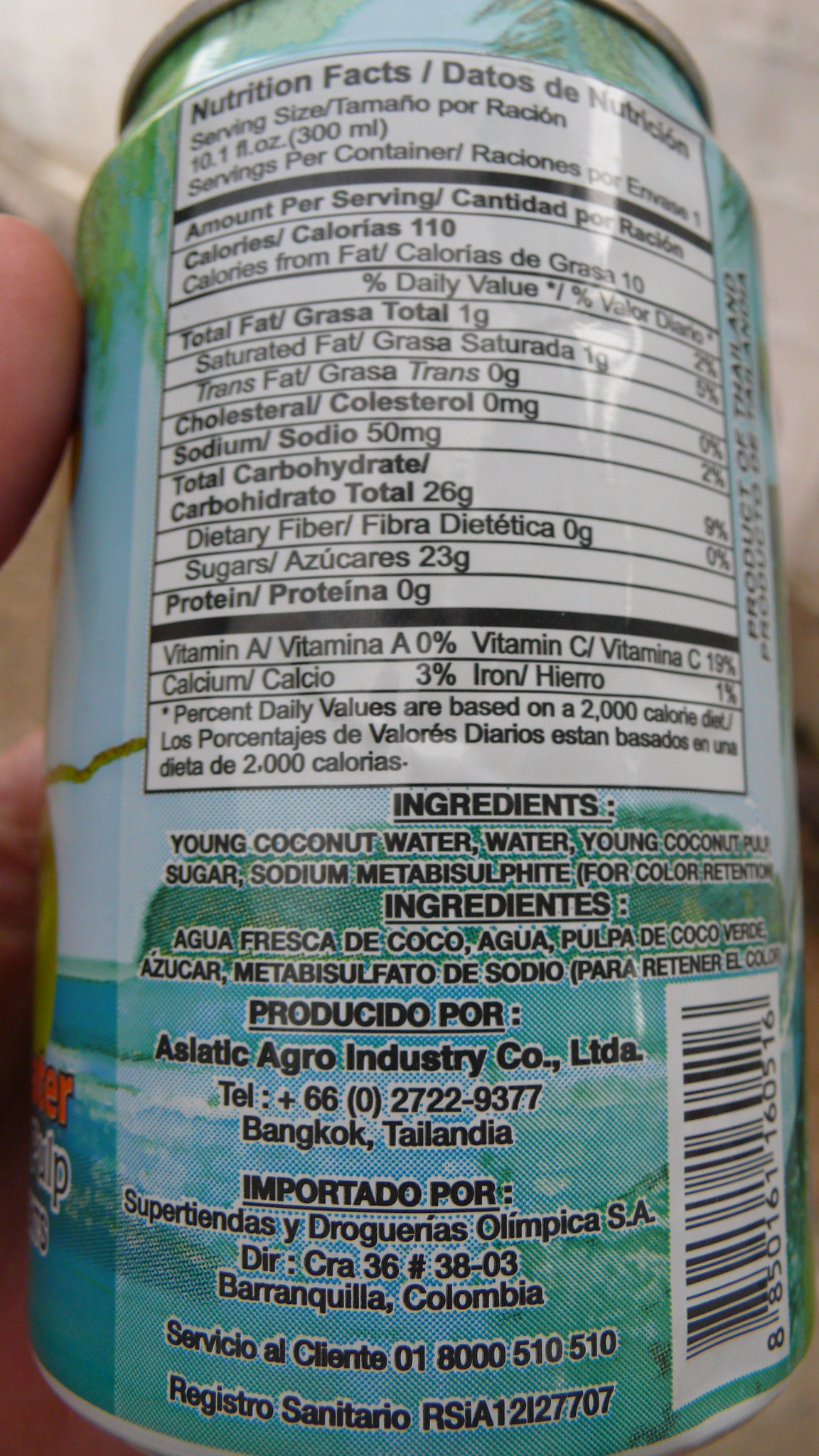**Detailed Caption:**

The image depicts a can filled with young coconut water. The can's design features a serene scene portraying a clear blue sky and a vast expanse of blue water, with a small green island visible in the background. On the bottom right corner, a barcode is situated for product identification. The label asserts that it is a product of Thailand.

The ingredient list is meticulously detailed, disclosing that the contents include young coconut water, young coconut pulp, sugar, and sodium metabisulfite, which is used for color retention. This information is also presented in Spanish, noting "Agua fresca de coco, agua pulpa de coco verde, azúcar metabisulfito de sodio para mantener color."

Additionally, the can mentions the manufacturer, Rhodosil By Athl, and the company Agro Intricol Limited. Contact information is provided: telephone number +66 2722-9377, located in Bangkok, Thailand. The product is imported and described as an important asset for "super tinnity." The bottom section contains some unclear information, possibly referencing import codes or batch numbers: "T-I-R-C-R-A 36 pound, 38 to 3."